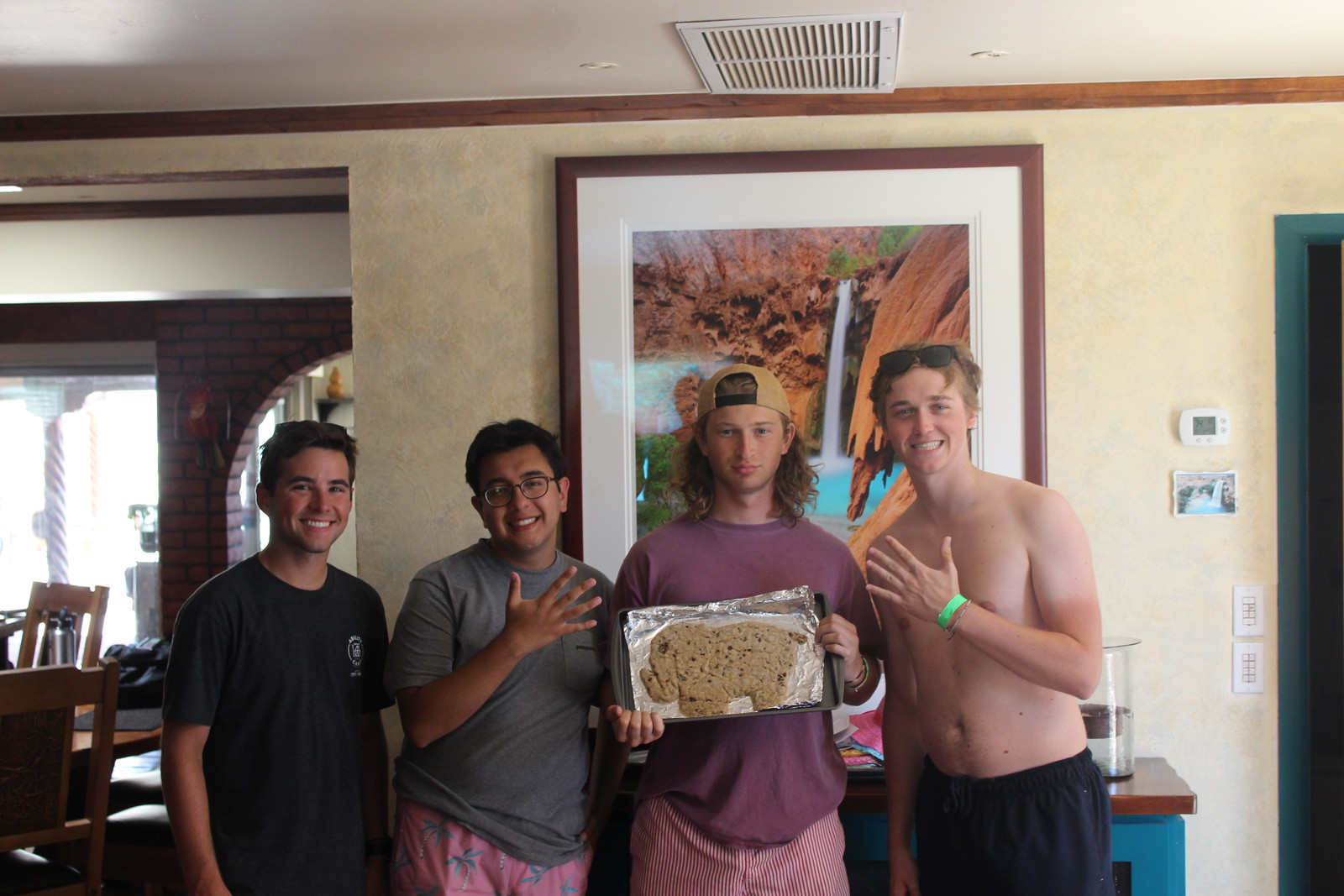This image features four young males standing side-by-side in a living room. The middle person, wearing a pinkish shirt and a backwards hat, is holding a baking sheet with cookie dough shaped like an elephant and covered in tinfoil, facing the camera. To his left (the right side of the image), a young male stands shirtless with black pants, glasses perched on top of his head, and a smile on his face. On the tray-holder’s right (the left side of the image), another young male with a gray shirt, pink pants adorned with tree designs (likely palm trees), glasses, and dark hair, stands smiling, with his hand up. The person at the far left is wearing a dark, short-sleeved shirt and is also smiling. Behind them, a picture of a waterfall in a wooden frame hangs on a beige wall. Additional details in the room include a table, chairs, sunlight, and an air-conditioned or vented ceiling.